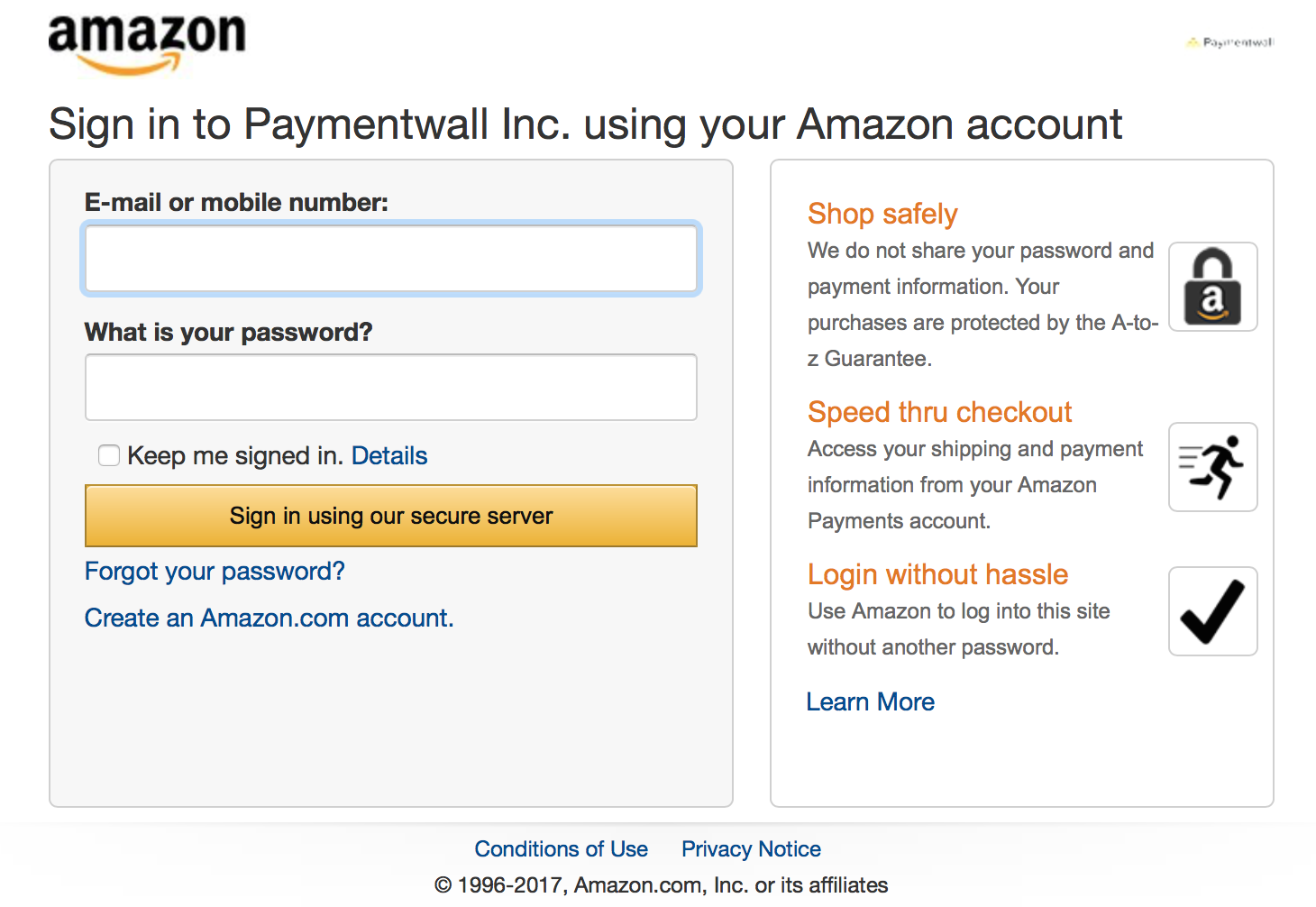The image is a screenshot of an Amazon sign-in page, prominently displaying the typical login credentials fields for entering either an email address or a mobile number, followed by the password field. This page is associated with PaymentWall Inc., which allows users to sign in using their Amazon account, facilitating a seamless login experience without the need to remember an additional username and password specific to PaymentWall.

At the top, the page prompts users with the text "Sign in to PaymentWall Inc using your Amazon account." This indicates that the user is on the PaymentWall site and intends to log in using their Amazon credentials for convenience.

To the right side of the login form, there is a section highlighting the benefits of using an Amazon account for the sign-in process. This section includes three key points, each accompanied by a relevant icon:
1. "Shop Safely" – Depicted with a padlock icon featuring the Amazon logo, indicating secure transactions.
2. "Speed through Checkout" – Illustrated with an icon of a person running swiftly, symbolizing expedited purchasing.
3. "Log in without Hassle" – Represented by a checkmark, denoting ease and efficiency in the login process.

These benefits are emphasized with orange text to capture the user's attention, reinforcing the advantages of utilizing Amazon's account services for a smoother and safer shopping experience on PaymentWall.